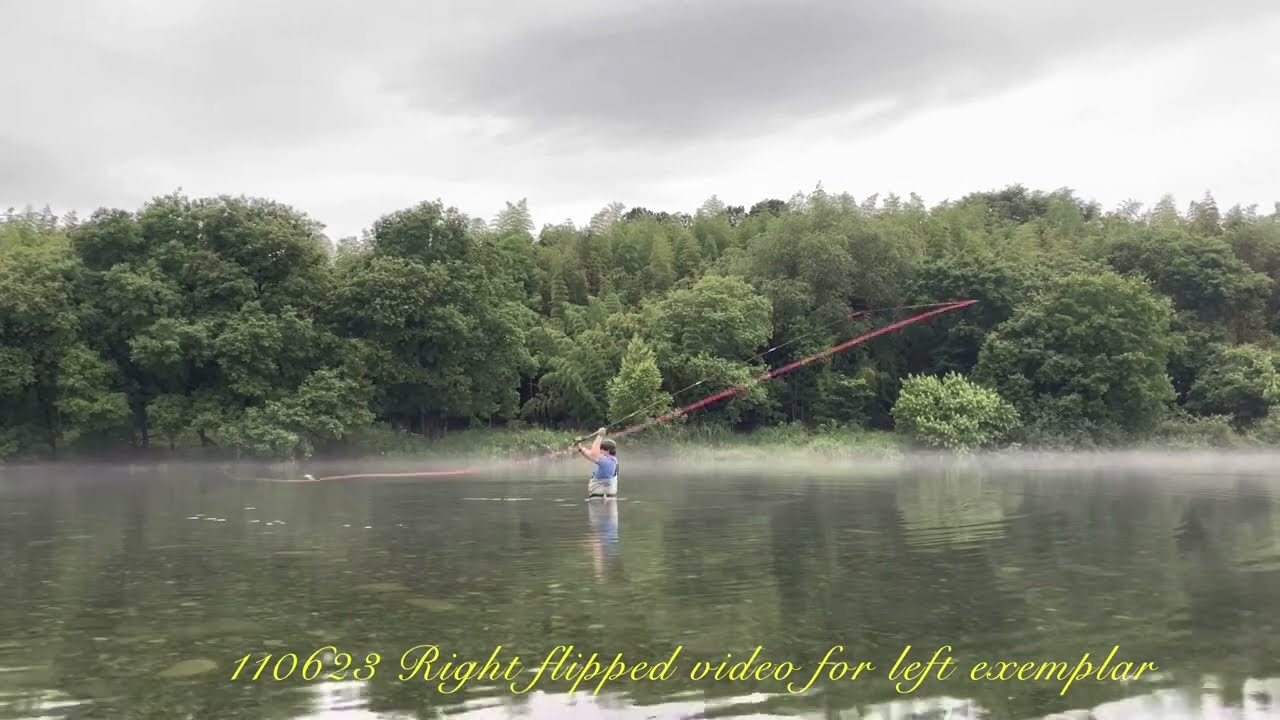The image depicts a man standing waist-deep in murky, greenish-brown water, likely a lake or pond, surrounded by lush, green trees in the distance. He is clad in blue t-shirt and fishers' waders, which have suspenders extending up to his chest, suggesting he is prepared to keep dry while in the water. The man, appearing to have brown hair, is holding a long fishing rod that looks pink or red. Above, the sky is overcast with gray and white clouds reflecting off the water’s surface. The image is notable for the yellow, metallic cursive text at the bottom which reads, "110628 right flipped video for left exemplar."